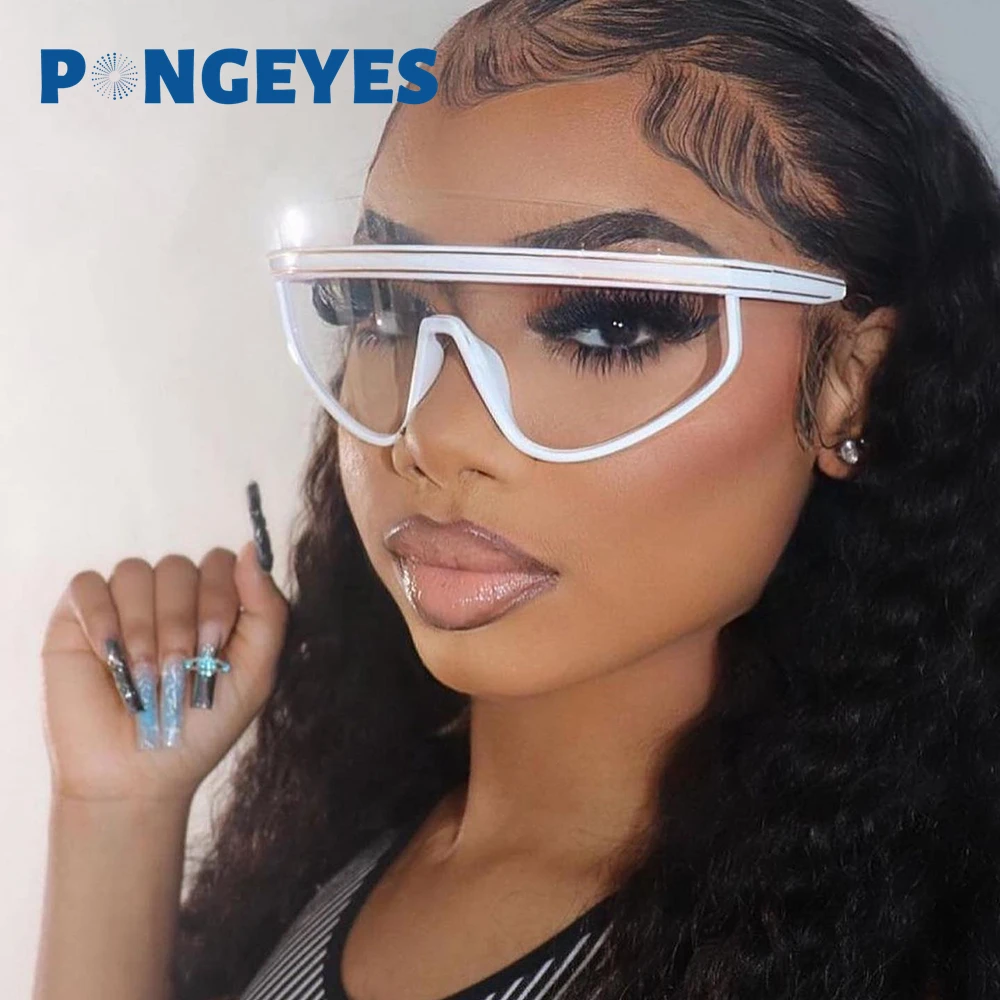This striking close-up photograph showcases an African-American female model with long, wavy, slightly frizzy dark hair. She dons oversized, futuristic white-rimmed glasses with clear, plexiglass-like lenses by the brand Pong Eyes (P-O-N-G-E-Y-E-S). Her makeup is meticulously done, featuring stud earrings, fake eyelashes, eyeliner, eyebrow liner, lip liner, and bold lipstick accentuating her pouty lips. She is dressed in a stylish black and white ribbed top with a black collar, complemented by her long, black and blue sparkly fake nails. The model is slightly angled to the left, perfectly capturing her expression and the detailed design of her accessories.